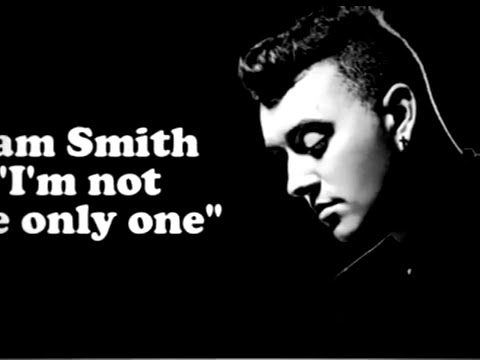The image is a highly stylized black-and-white photograph of Sam Smith. Set against a completely black background, the photograph prominently features Sam Smith on the right side. His head is turned to the left, and he gazes downward, his eyes closed or downcast, adding a contemplative aura. Smith's hair is cut short and comes into a sharp widow's peak, with a slightly tufted top. He has angular facial features, with thick eyebrows, a pointed nose, and closed lips, giving a serene yet intense profile. He appears to be wearing a black jacket or shirt, which blends into the shadows, rendering the details indistinct. A small ear stud is visible. 

To the left of Smith's face, in large white block letters, are fragmented words intended to read: "SAM SMITH, I'M NOT THE ONLY ONE," presented in quotation marks. However, due to the layout, only segments of the text are fully visible, appearing as "AM SMITH," "I'M NOT," and "E ONLY ONE," with portions of letters cut off at the margins, abstractly teasing the full phrase. The contrast between the stark black background and the bright white text amplifies the minimalist yet striking visual impact of the photograph.